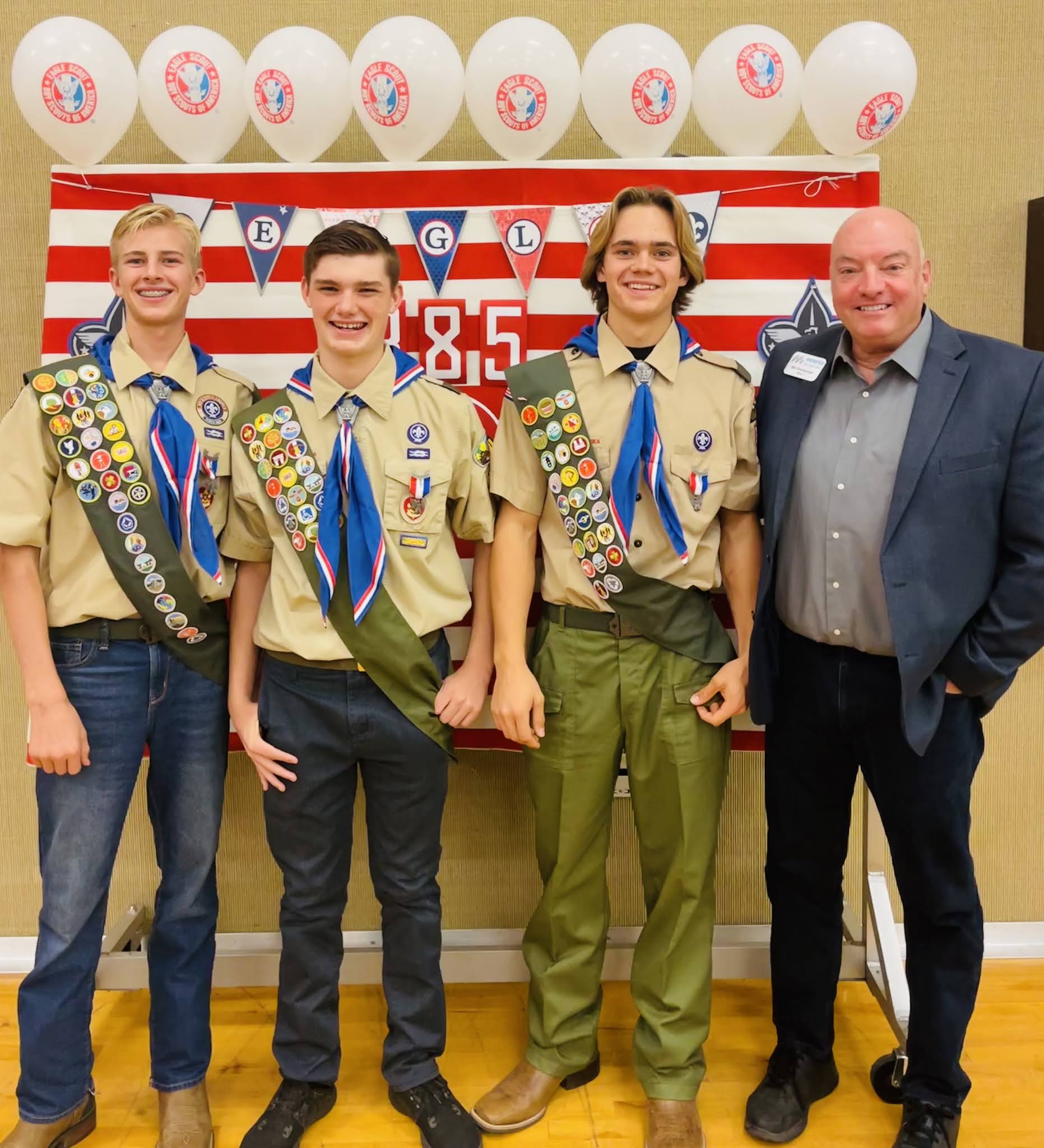This full-color, vertically rectangular photograph, taken indoors with artificial lighting, captures a memorable Boy Scouts of America event. The setting features a light wood floor with white floorboards against a brown wall, and several white balloons adorned with the Boy Scouts of America logo. A red and white banner, showing the number 85, hangs prominently in the background.

Posing proudly in the image are four individuals: three high school-aged Boy Scouts and an older, bald gentleman in a blue suit jacket. The three Scouts, estimated to be around 16 years old, wear their official Boy Scout shirts. Two of them are dressed in blue jeans, and the third in traditional Boy Scout pants. Each Scout sports a blue neckerchief accented with red and white stripes, and across their chests, they wear green sashes heavy with merit badges. Over their rank patches, be it Eagle Scout or Life Scout, they display red, white, and blue ribbons with medallions—a testament to their achievements.

The older gentleman, standing to the right of the Scouts, complements their attire with his suit jacket and name tag on the lapel, symbolizing his role in the ceremony. Together, they form a proud tableau that celebrates the accomplishments and camaraderie of the Boy Scouts of America.